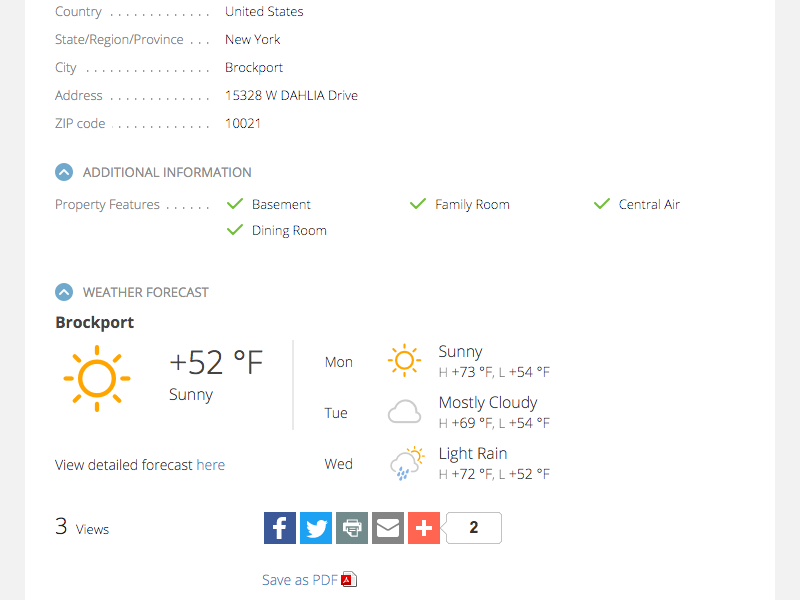This image is a detailed screenshot of a weather report for Brockport, New York, USA. In the top left corner, the report specifies the exact location as 15328 West Delilah Drive with the ZIP Code 10021. Additionally, it provides property details, indicating that the house features a basement, a dining room, a family room, and central air conditioning. The bottom section of the page displays the current weather conditions: Brockport is enjoying a sunny day with a temperature of 52 degrees Fahrenheit, symbolized by an accompanying sun icon. To the right, a three-day forecast is provided, showing sunny weather on Monday, mostly cloudy skies on Tuesday, and light rain on Wednesday. At the very bottom of the screenshot, there is a blue link that reads "Save as PDF."